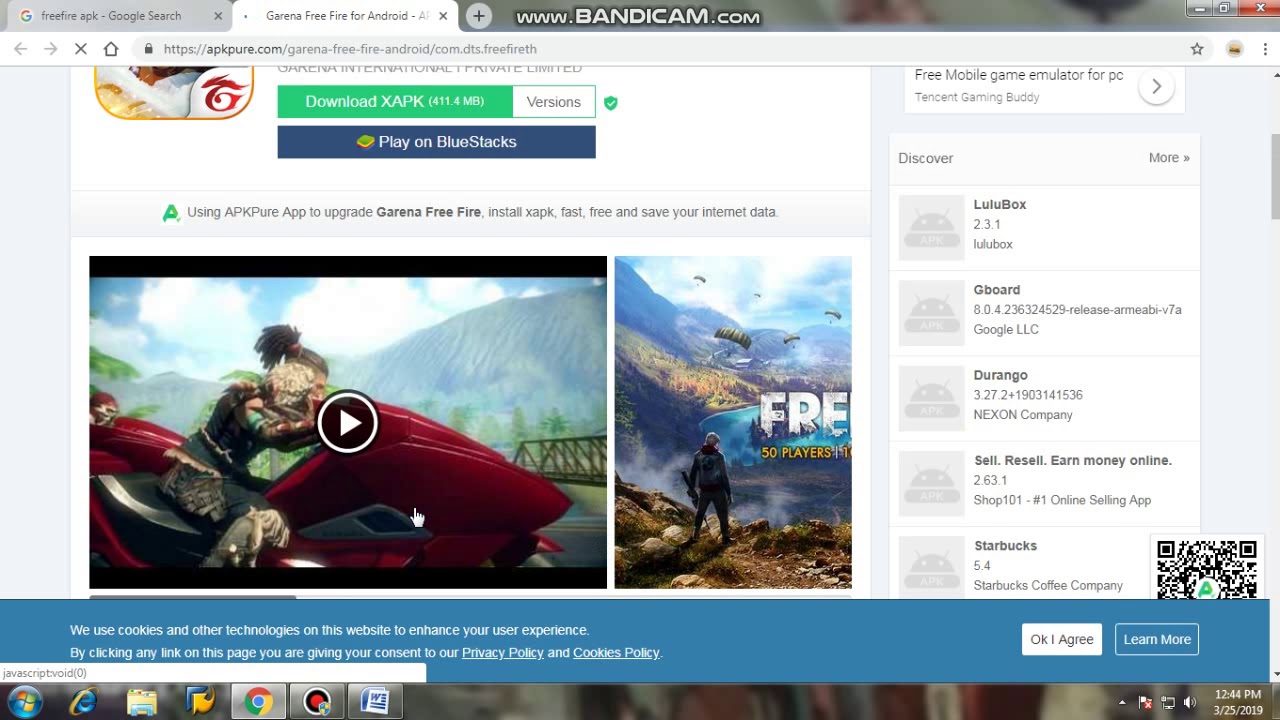This is a detailed screenshot of a desktop running Windows, likely Windows 8 or 10, as evidenced by the characteristic taskbar at the bottom of the screen. The Windows taskbar includes various icons typical of the operating system. 

Displayed prominently on the desktop is a Google Chrome browser window with two open tabs. The current tab is actively engaged with the URL bar showing the address: "apkpure.com/garena-free-fire-english.com.dts.freefire-th". Adjacent to this tab, another tab is open with the address: "www.bandicam.com".

The visible webpage on the open tab appears to be a download page for an application, most likely the game "Garena Free Fire". Scrolling down slightly within the browser reveals a prominent green download button labeled "Download .XAPK (411.4 MB)". Below this green button is a secondary blue button labeled "Plan BlueStacks". Additionally, under these buttons, there is an embedded video related to the download content.

The layout and elements of this webpage suggest it is designed for facilitating user downloads and providing supplementary information via the video content.